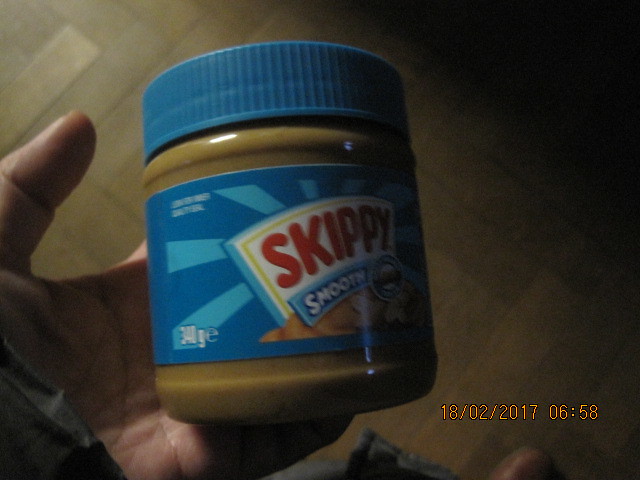This color photograph, possibly taken with a cell phone or digital camera, captures a person's left hand holding a small, full jar of Skippy Smooth peanut butter. The hand, positioned on the left side of the image, reveals only the thumb and fingertips, partially obscured by the jar. The Skippy peanut butter jar features a blue textured lid matching the dark blue and light blue label. "Skippy" is prominently displayed in red rounded font on a white rectangular background, while "Smooth" is written below in white font with a blue outline on a light blue background. The background reveals a dark wooden or faux wood floor and the tip of a brown boot shoe at the bottom right. The photograph is marked with a date and time stamp reading "18-02-2017 06:58." The image is somewhat blurred and dimly lit, with slight illumination on the hand. There is no other writing or visible subjects apart from the described elements.